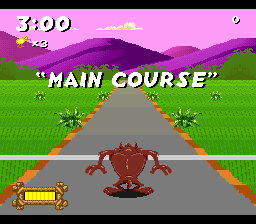In this video game screenshot, the scene is set under a light purple sky dotted with a single white cloud, and framed by deep purple mountains. At the bottom, a gray runway stretches into the distance, labeled "Main Course" in white text and quotation marks. The runway is flanked by vibrant green grass on both sides, with its outer edges bordered by vertical patterns of light brown and dark brown rectangles. 

At the top left corner of the image, there is a timer displaying "3:00". Directly below the timer is a yellow icon followed by the text "x3". To the right of this, a small number "0" is displayed. The focal point of the image is a short, brown character viewed from the back. On the left side of the screen, there is a vertical bar framed in brown containing a yellow progress bar.